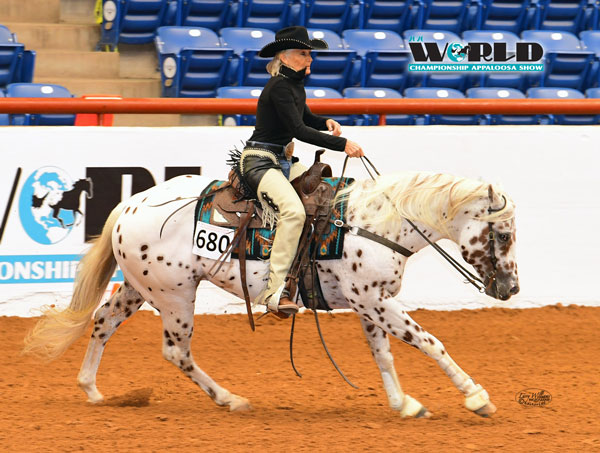In the foreground of this detailed image, we see an elderly woman with a grayish blonde ponytail riding a beautifully spotted horse on the reddish-brown dirt floor of an outdoor stadium. The stadium's blue seats climb high into the background, with visible stairs interspersed between the seating areas. The woman is dressed in a black cowboy hat and a black long-sleeved shirt or turtleneck, paired with distinctive white chaps that feature black fringe. Her tan pants peek out from under the chaps. Her right hand is gripping the horse's bridle, while her left hand is raised confidently in the air, suggesting she's in the midst of a performance or competition.

The horse she rides is striking, marked with Dalmatian-like white and black speckles concentrated particularly on its face. The horse sports a blonde mane and tail and is equipped with a brown saddle adorned with turquoise accents and the number 680, hinting at its participation in the event. The saddle is complemented by a matching blanket underneath. 

To the top right of the image, the logo for the "World Championship Appaloosa Show" is prominently displayed, with a globe representing the 'O', further indicating the competitive nature of the scene. The dynamic stance of the horse, with dirt kicking up behind its back legs, captures the moment of its steady movement.